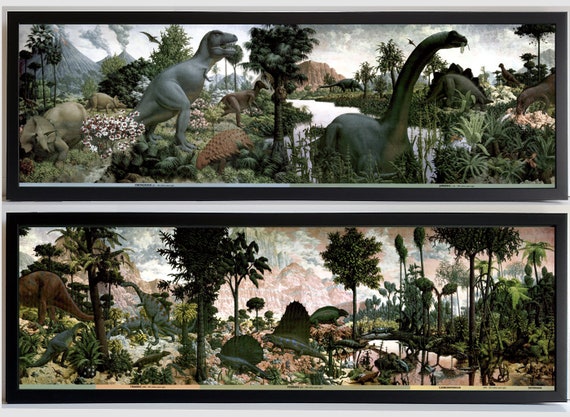The image consists of two detailed drawings of dinosaurs positioned one above the other. The upper drawing showcases a prehistoric landscape featuring several dinosaurs amidst abundant greenery and natural elements. From the upper left, volcanoes billow with smoke, setting a dramatic background. Below the volcanoes, a beige-colored dinosaur stands, while to its right, a larger gray dinosaur occupies a significant portion of the image. Behind and below these creatures is a lush, green environment filled with various trees and vegetation. Further to the right, an even larger dinosaur of a darker gray hue appears, with a small river flowing behind it and more dinosaurs and shrubbery extending to the right.

The lower drawing mirrors the vivid detail of the upper one but with a notable difference in scenery. This second image also features dinosaurs and dense shrubbery, but the background prominently includes mountainous regions, which are depicted in orange and brown hues, contrasting the dominant green tones of the foliage. Together, the drawings create a vibrant and comprehensive depiction of a prehistoric world teeming with diverse dinosaurs and dynamic landscapes.